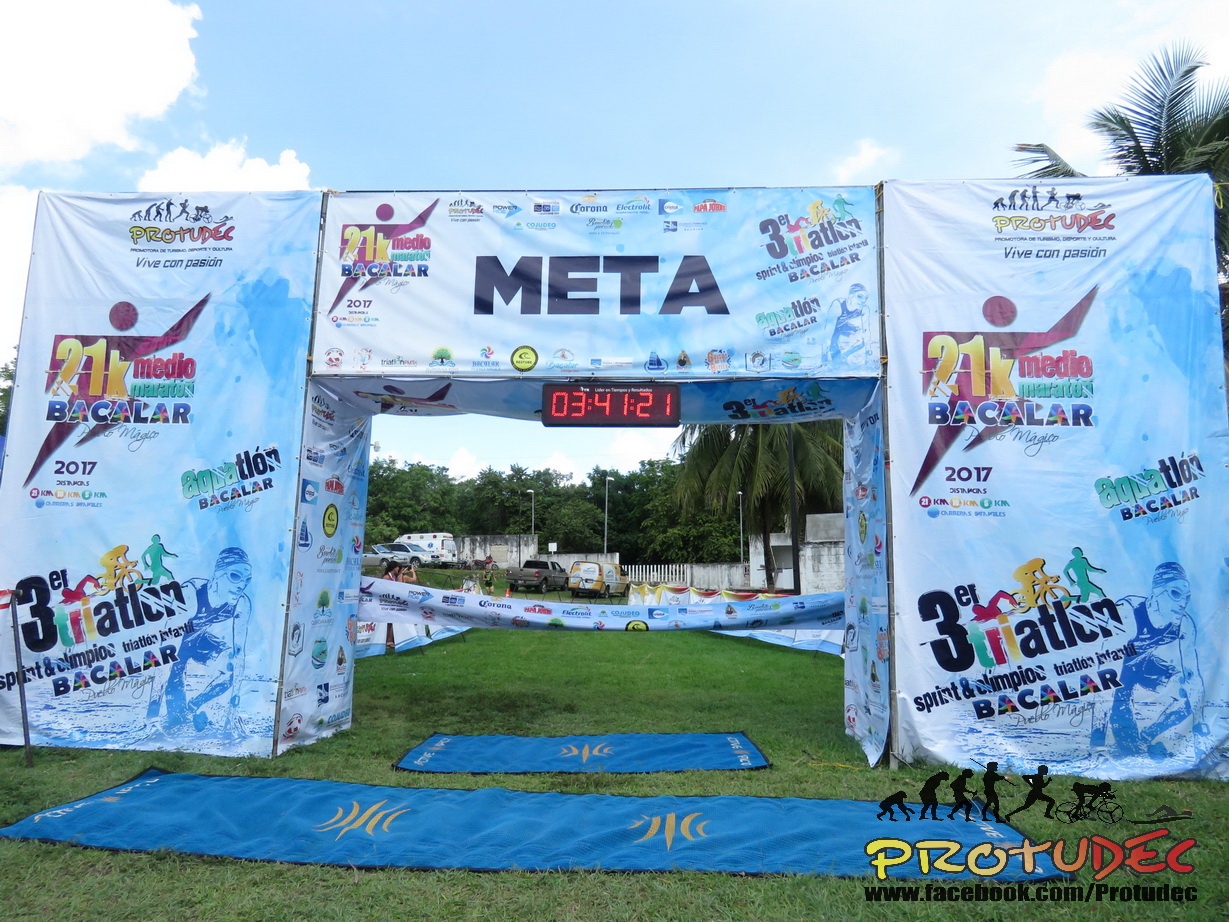The photograph captures an outdoor race event, likely a triathlon, set in a grassy area under a partly cloudy sky. The focal point is a large finish line structure composed of two vertical pillars connected by a horizontal beam, covered in a bluish-white fabric with various graphics. Prominently displayed in the center is the word "Meta" in big black letters, beneath which a digital stopwatch reads "03:41:21," indicating the time for the competitors crossing the line. Surrounding the finish line and scattered on the grass are several tarps, and numerous people are seated on the ground. Behind them, cars are parked along a fence lined with trees. The finish line structure also features images of a runner and mentions "21K Bacalar" and "3EI," signifying the race's association with Bacalar. Additionally, it showcases various sponsors' logos, including "Pro True Deck," and a graphic silhouette representing the evolution from ape to running man, culminating in a cyclist.